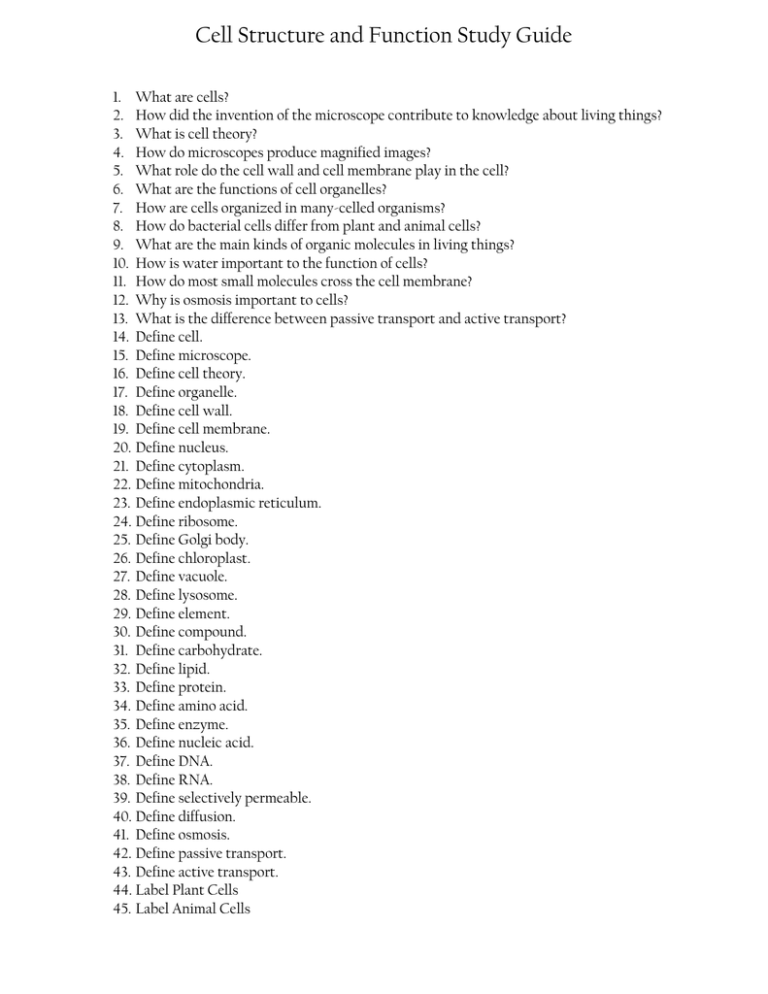The image features a stark white background with text organized in a structured format. At the top of the image, in bold black letters, the title "Cell Structure and Function Study Guide" is prominently displayed. Below this header, there is an extensive list of 45 questions numbered consecutively from 1 to 45, each written in small black font. The questions encompass a broad range of topics related to cell biology, including foundational concepts and definitions. For example, the questions cover basic inquiries such as "What are cells?" and "What is cell theory?" to more detailed questions like "What role do the cell wall and cell membrane play in the cell?" and "How do bacterial cells differ from plant and animal cells?"

Moreover, the list delves into the functions and definitions of various cellular components and organic molecules, addressing elements like the nucleus, mitochondria, Golgi body, and chloroplasts. It also differentiates transport mechanisms such as passive and active transport and highlights the importance of water and osmosis in cellular function. Each question aims to build a comprehensive understanding of cell structure and function, exemplified by requests to define specific terms including "amino acid," "enzyme," "DNA," and "selectively permeable." The list culminates with tasks to label both plant and animal cells, suggesting a visual component to the study guide. Overall, the setup is clear and organized, designed to facilitate a thorough review of cell biology concepts.